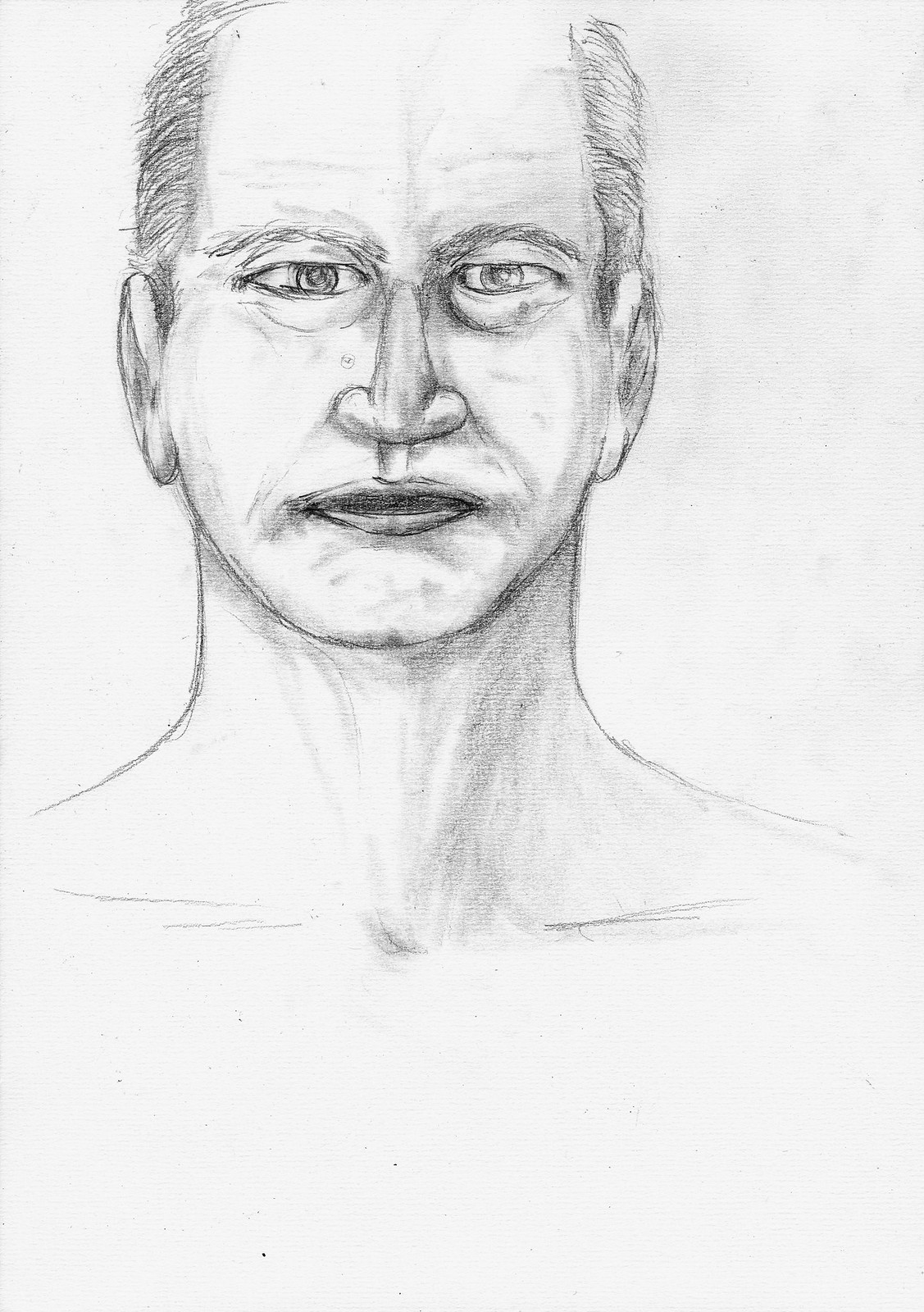This black and white, portrait-format pencil sketch depicts a serious-looking man, likely in his 40s, with a clear focus on realistic detail, despite not being perfectly executed. The man has a large forehead with thinning hair swept back, suggesting age or early signs of balding. His rounded chin, large nose, and closely set, prominent ears frame a face marked by heavy bags under his eyes. Horizontal wrinkles traverse his forehead, and there's a noticeable dot beside his nose. His thick neck leads to visible collarbones, hinting at an unfinished torso stopping above the shoulders. The background is shaded grey, and overall, the portrait illustrates the artist's evident experience in sketching, even as they strive for realism with varying success.